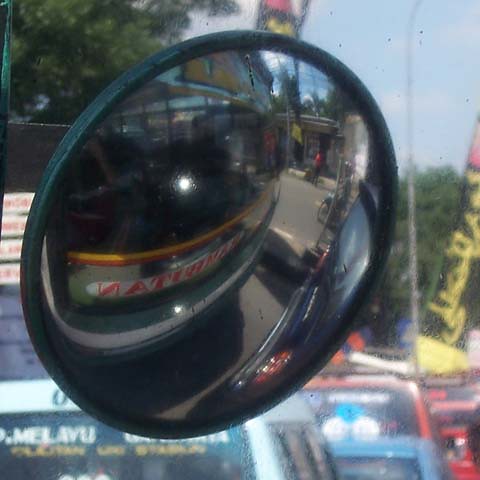Captured in this photograph is a circular, fish-eye style domed mirror installed inside a bustling city bus. The mirror, designed for the bus driver to monitor approaching passengers, is securely mounted on the glass interior of the bus. The scene outside the bus reveals a congested city street, with numerous rows of cars suggesting a busy urban environment. The glass to which the mirror is attached shows visible imperfections and spots of dirt, adding a sense of realism to the everyday hustle and bustle captured in the image.